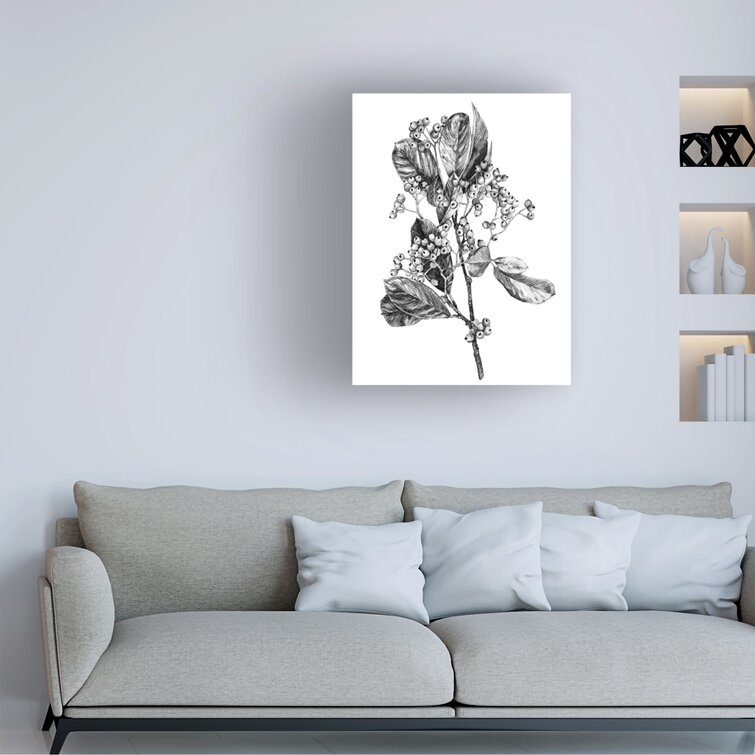The photograph captures an indoor living room scene, centered around a wall adorned with art and shelving. At the bottom of the image, a modern, gray couch occupies approximately one-third of the frame horizontally. The couch features a low profile and is divided into two sections; it has two main cushions and is accented with four light gray throw pillows, with three pillows positioned on the right and one on the left. Above the couch, a frameless rectangular painting commands attention. The painting has a minimalist white background showcasing a black and white depiction of a plant with leaves and berries. To the right of this painting are three built-in wall shelves. The shelves display an assortment of items: a black art installation on the top shelf, a white art piece in the middle, and white objects resembling books on the bottom shelf. The wall itself is painted a light gray, contributing to the calm, cohesive aesthetic of the room.